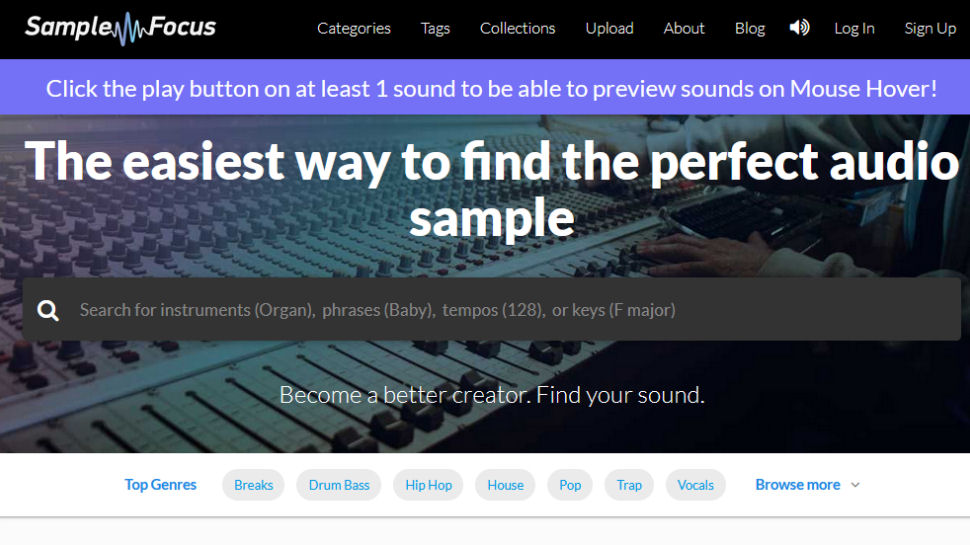The web page features a sleek black header with white text, prominently displaying the logo "Sample Focus" in the top left corner. The logo includes a distinctive sound wave graphic that creatively connects the letters 'E' and 'F'. To the right, you'll find navigational links labeled "Categories," "Tags," "Collections," "Upload," "About," and "Blog." Additionally, there are icons for sound and user account management, with options to "Log In" and "Sign Up."

Directly beneath the header, a purple bar with white text advises users: "Click the play button on at least one sound to be able to preview sounds on mouse hover." Below this advisory, the main feature area showcases an image of a professional soundboard, typically used in music mixing, providing a visually relevant backdrop.

Overlaying the soundboard image, bold white text headlines the section, stating: "The easiest way to find the perfect audio sample." Beneath this headline is a gray search bar prompting users to "Search for instruments (e.g., organ), phrases (e.g., baby), tempos (e.g., 128), or keys (e.g., F major)."

The section continues with a tagline in smaller white text: "Become a better creator. Find your sound." Further down, a white bar featuring blue text introduces "Top Genres," which includes buttons for popular categories like "Breaks," "Drum & Bass," "Hip Hop," "House," "Pop," "Trap," and "Vocals." There is also a "Browse more" button with a drop-down arrow for additional options.